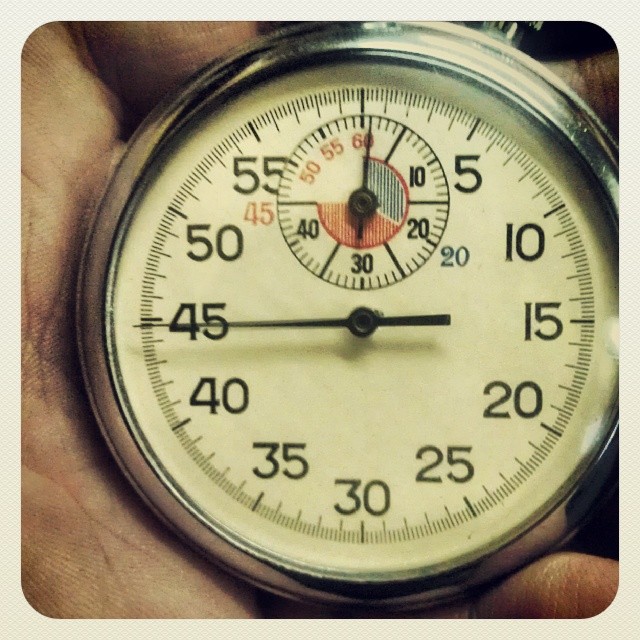A very close-up image captures a stopwatch held in someone's hand. The left side of the image reveals the subtle contours of the person's palm, while the bottom right corner hints at a finger, though fine details remain indistinct. The stopwatch, a shiny, bright silver, is prominently featured at the center. Its round face boasts a light, creamy-yellow hue, with black numerals clearly marking the time. The main display appears to be stopped at 44 seconds. Above the main hands, there's a smaller circular dial with a touch of red, and its hand points to 60, though its specific function is unclear. The hand holding the stopwatch is light in complexion, with a noticeable pinkish-white tone enhancing the bright silver encasing of the stopwatch.